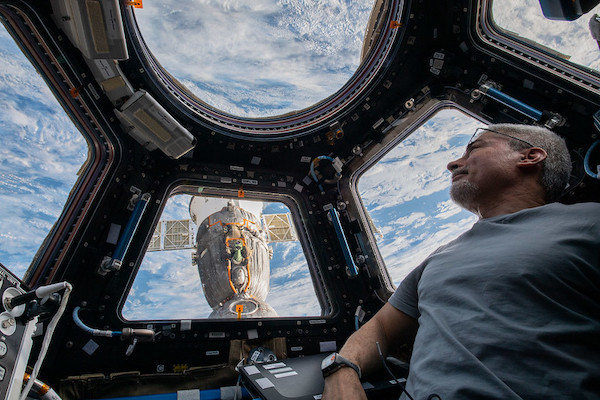The photograph captures a detailed scene inside a space shuttle, focusing on a man positioned in the lower right corner, visible from the waist up. This man, wearing a grey t-shirt and glasses, has short grey hair and a grey goatee and wears a black wristwatch on one arm. He is intently looking up through a circular window, one of several aboard the shuttle. The shuttle's interior, which features numerous tubes, cables, controls, and a closed laptop that the man appears to lean on, suggests a highly technical environment. The windows have black frames, with unique shapes—parallelogram windows tapering from narrow at the top to wide at the bottom. Through these windows, one can see the vibrant blue of Earth's atmosphere, dotted with white clouds, and an external satellite with grey, orange, and green parts. The man appears to be observing the Earth and its atmosphere, emphasizing the altitude and perspective of space travel.